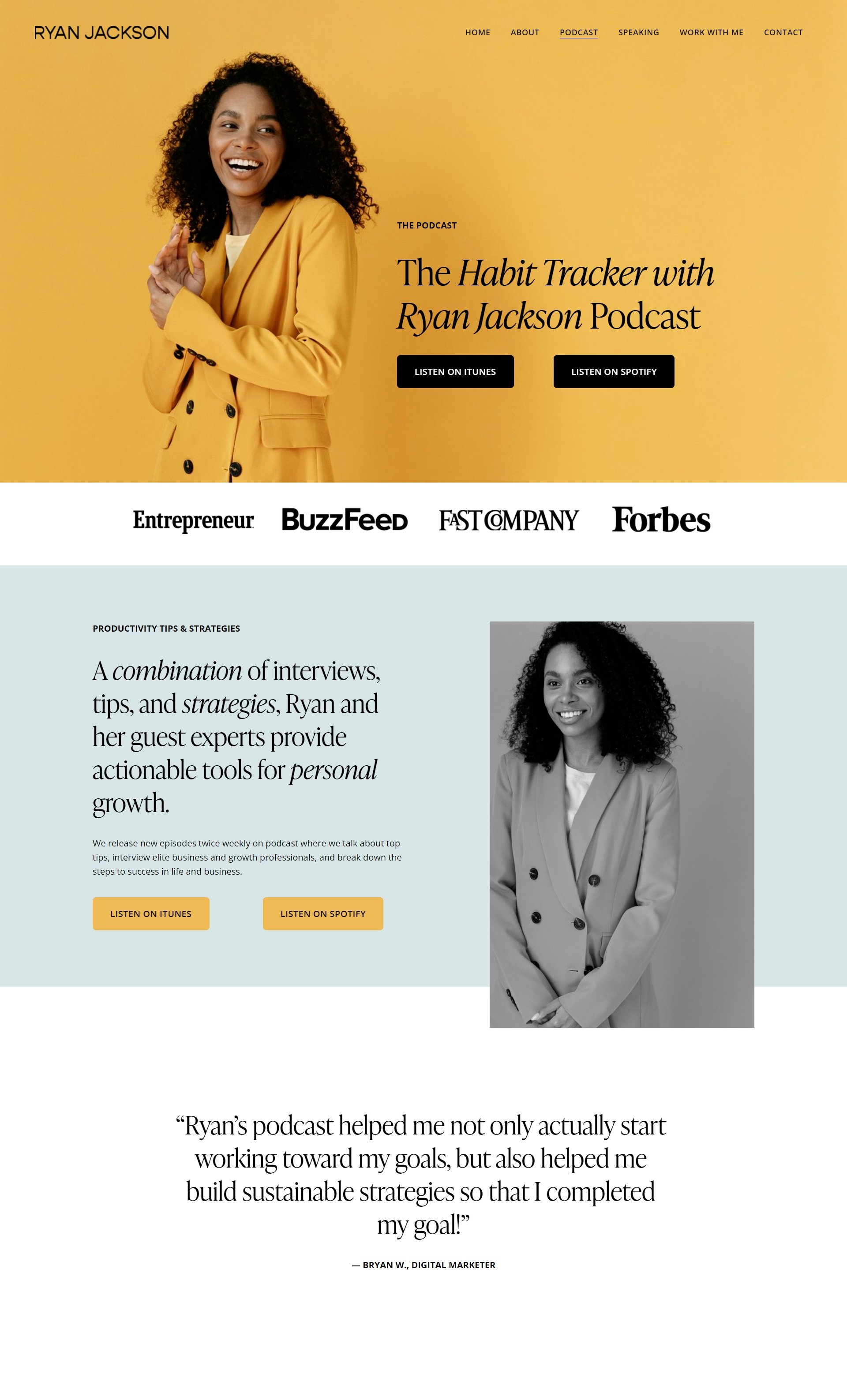**Detailed Caption:**

The image features a vibrant advertisement for the "Ryan Jackson Habit Tracker Podcast" hosted by Ryan Jackson, designed to capture the attention of individuals seeking personal growth and self-betterment. The focal point of the webpage showcases a light-skinned Black female, identified as Ryan Jackson, donning a bright yellow sweater against a matching yellow background, exuding positivity and warmth.

At the top of the page, bold black text on a vivid yellow backdrop introduces the podcast as a comprehensive resource combining interviews, practical tips, and strategies. Ryan Jackson, along with her expert guests, delivers actionable tools aimed at fostering personal development.

Prominently displayed are two CTA buttons urging visitors to "Listen to the Podcast," complemented by another call to action in stark black and white contrast, ensuring visibility and emphasis on engagement.

In the midsection, a banner highlights endorsements from reputable sources such as Entrepreneur, BuzzFeed, Fast Company, and Forbes, underscoring the podcast's credibility and influence.

Further down, a green background segment reiterates the podcast's core offering— a blend of interviews, tips, and strategies—accompanied by a black-and-white photograph of Ryan Jackson in the same recognizable yellow sweater, strengthening brand consistency.

The advertisement wraps up with a powerful testimonial from a listener, lauding the podcast for not only motivating them to initiate action towards their goals but also for providing a structured strategy to achieve them. This affirmation is positioned strategically at the bottom, leaving a lasting impression of Ryan Jackson's life-enhancing podcast.